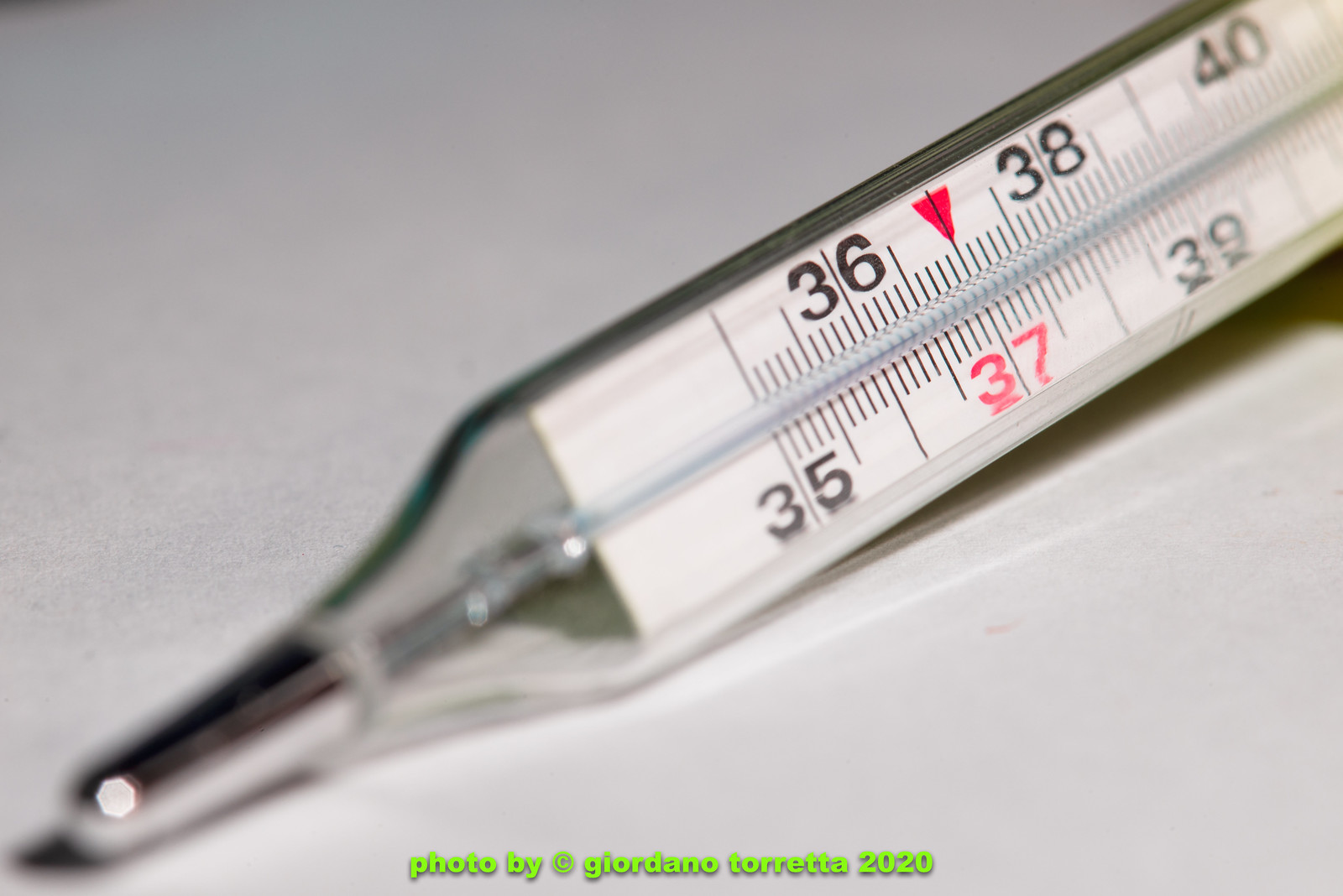The image features a close-up view of a thermometer set against a gradient background that transitions from gray in the upper left corner to a light gray or white in the lower right corner. The thermometer has a silver end, designed for oral use, extending into a glass tube. Inside the glass, a white scale is marked with black numbers: 35, 36, 38, 39, and 40. Between the numbers, there are longer lines where the numbers are and shorter lines in between. A red arrow pointing diagonally downwards to the right highlights the number 37, which is also written in red. The thermometer casts a shadow to the right and slightly below it. At the bottom of the image, green text reads "Photo by @GiordanoTorretta, 2020."